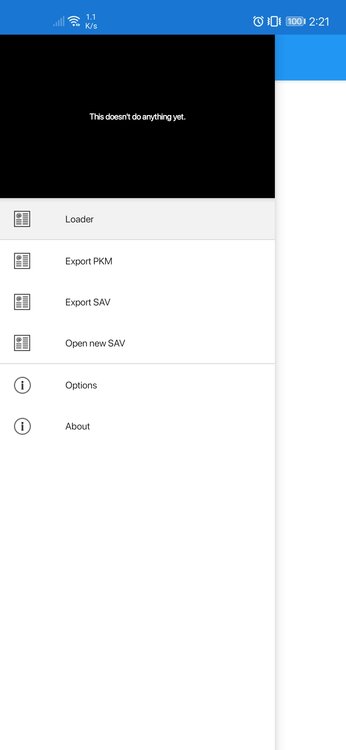This is a detailed screenshot from an Android smartphone. The notification bar at the top is blue and displays several icons: the time on the right, reading 2:21, a battery icon indicating 100%, and the Wi-Fi and phone signal icons towards the left. Below the notification bar, a dropdown menu is open against a white background. At the top of the menu, there's a black banner with the text "This doesn't do anything yet." Underneath this banner, there are four options, each accompanied by a similar icon. The options are: 

1. Loader (highlighted slightly darker)
2. Export PKM
3. Export SAV
4. Open New SAV

Below these options, there's a dividing line, followed by two additional options: "Options" and "About." The overall design of the app appears simple and clean, emphasizing functionality.